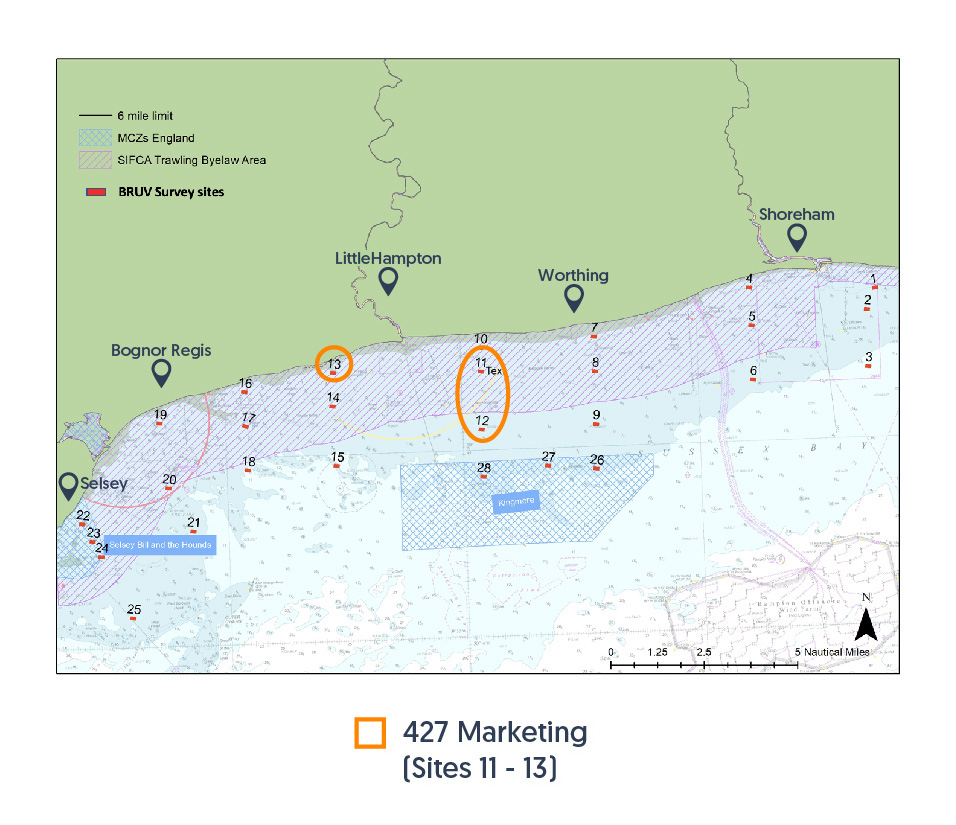The image appears to be a detailed survey map of a coastal region in England, used likely by professionals for tracking and locating various objects. The map features a 6-mile limit and includes designations such as "MCZs England" and "SIFCA Trawling By-law Area," indicating maritime conservation and regulations. Key marked sites include "Brew Site" and "Survey Site," denoting specific areas of interest. Significant locations labeled on the map are Worthing, Bognor Regis, Littlehampton, Shoreham, and Selsey, suggesting a focus on coastal towns. The map's upper portion is green, representing land, while the lower portion is blue and white, indicating water. Specific coordinates appear to track areas both onshore and nearshore. Additionally, it contains symbols and areas marked with diagonal lines and red squares, offering a detailed grid for precise navigation and surveying.